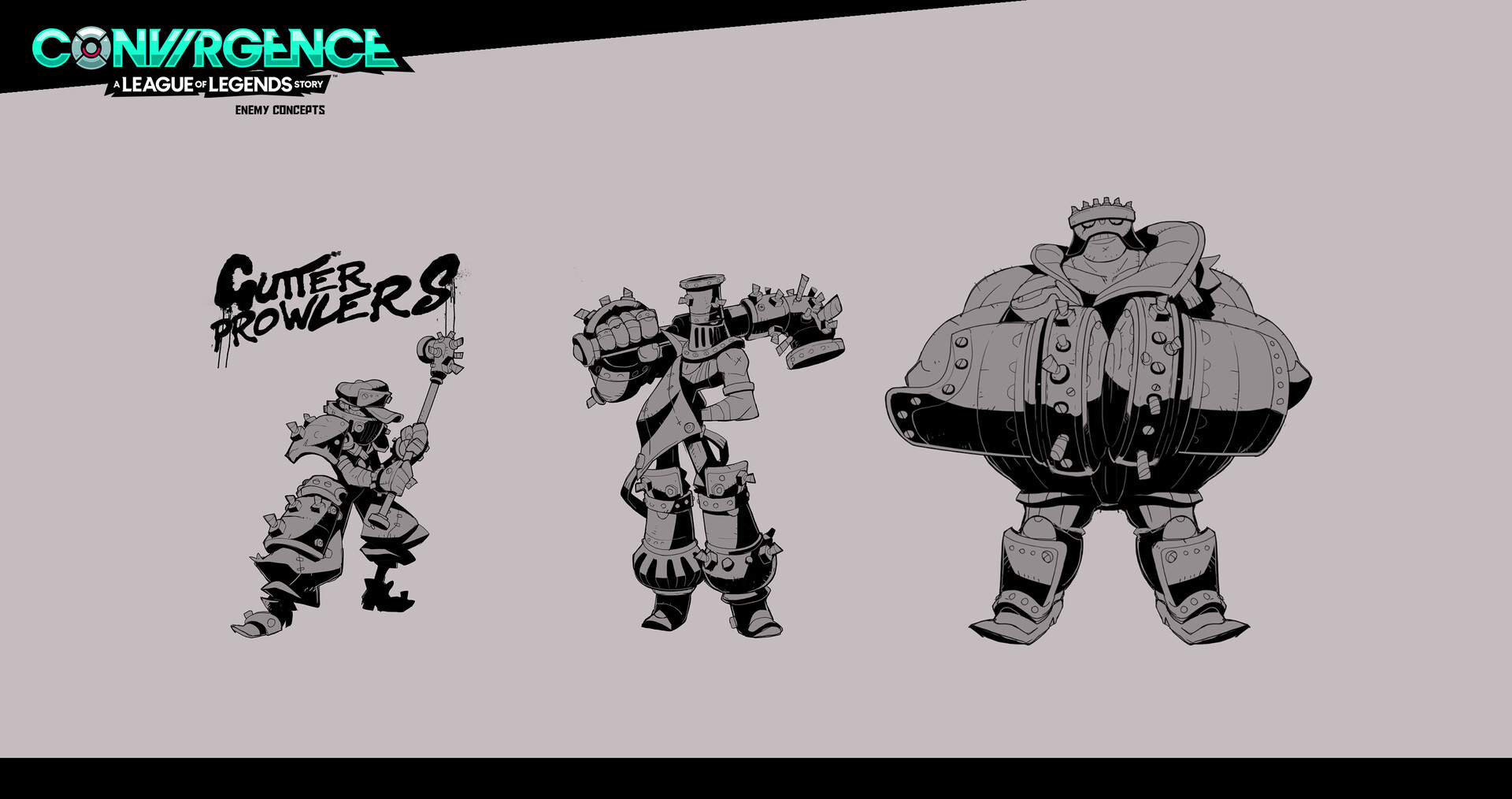The image is a detailed digital rendering, possibly a preliminary concept, featuring three fantasy characters set against a gray background. At the top left, in bright green, shiny letters, it prominently displays the title "CONVERGENCE, A LEAGUE OF LEGENDS STORY, ENEMY CONCEPTS." There's a noticeable dark strip at both the top and bottom of the image, acting as a framing element. On the left side, in a graffiti-like font, the text "GUTTER PROWLERS" is visible. The three characters are predominantly gray with black shading, giving them a metallic appearance. Each character is equipped with weapons made from pipes and gutter materials. The first character, on the left, appears to be completely gray and black, wielding a weapon. The center character looks like it's constructed from metal sheets and armor, holding a pipe over its shoulders. The character on the right is a towering figure with trashcan-like arms, broad armor, and sports a crown on its head, suggesting a position of authority or power among the trio.